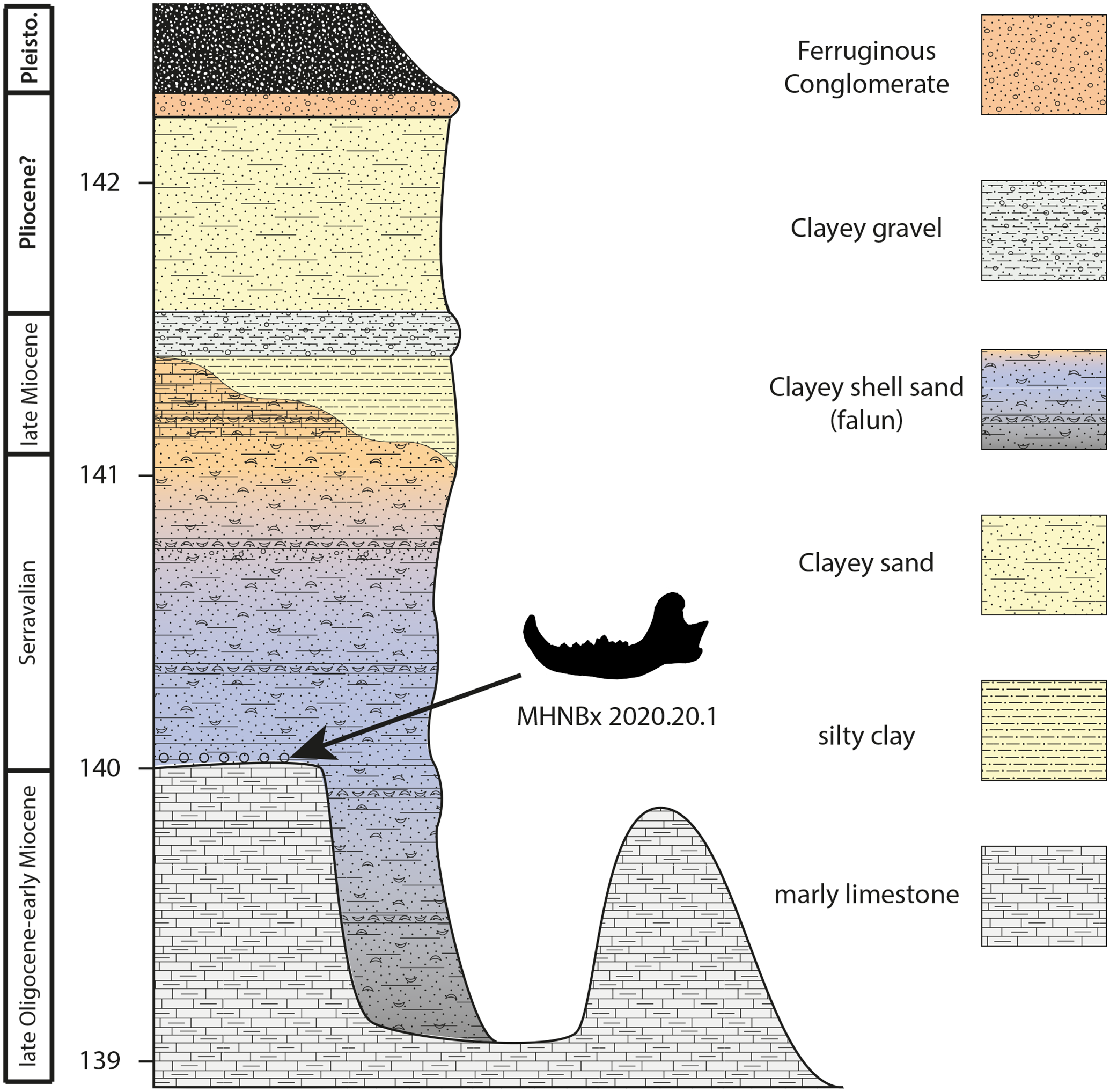The image is an informative geological chart, detailing various sedimentary layers with associated fossil findings. On the left side of the chart, there are numbered layers starting from 142 at the top and descending to 139 at the bottom. Each layer is identified by its type: Phryginia’s conglomerate (orange with black dots), clayey gravel (white with black dots), clayey shell sand (blue with black dots), clayey sand, silty clay, and marley limestone.

To the right, a colored drawing visually represents these sedimentary layers, aligning with the legend on the far right. The legend uses distinct colors to denote each type of sediment: a peach square for Phryginia’s conglomerate, white for clayey gravel, purple for clayey shell sand (falloon), light yellow for both clayey sand and silty clay, and white for marley limestone.

A prominent feature of the chart is a black jawbone fossil, highlighted with an arrow that points to its corresponding layer, providing a clear indication of where this fossil was discovered within the geological strata. The image combines textual descriptions and colorful visuals to effectively convey the distribution and types of sediments, emphasizing the locations where fossils like the jawbone may be found.